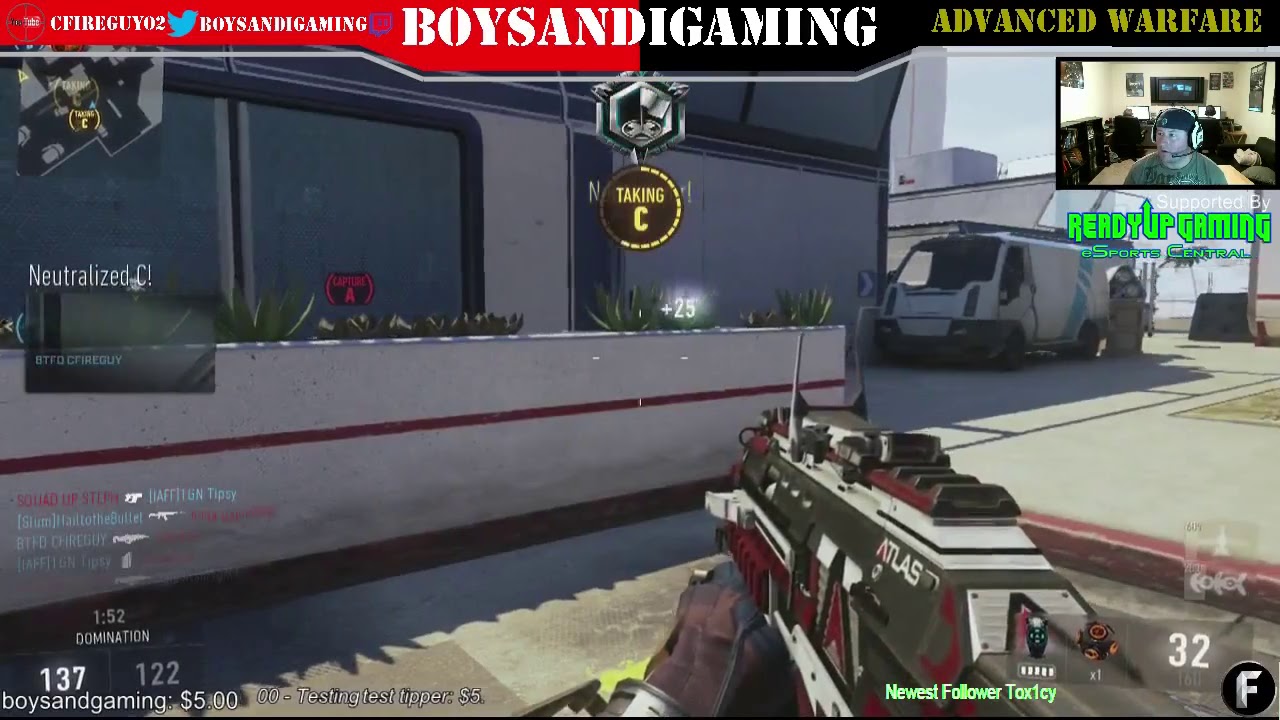This detailed screenshot from a video game, "Boys and I Gaming," features a complex mix of imagery and text overlays. At the top, there's a red and black background with white text displaying "Boys and I Gaming" alongside a Twitter handle, CFIREGUY02. To the right, "Advanced Warfare" is written in olive green. A logo of a blue dove is also present. The interface showcases various player statistics including a $5 tip indicator, and numbers 137 above 122, with a timer displaying 1:52 under the heading "Domination."

Central to the image, the player holds a red and gray "Atlas" gun, and the on-screen objective is "Taking C," noted in a circular area amidst a plaza. To the middle left, the phrase "Neutralized C!" is visible. The environment depicts a white van facing left, partially obscured by a wall with a red stripe and potted plants. On the right of the screenshot, there's a smaller window of a player wearing headphones, focused intently on the game, highlighted by the "Newest Follower" section on the bottom right, with the letter "F" in a black circle. The intricate scene combines realistic graphics and HUD elements, presenting an immersive gaming experience.